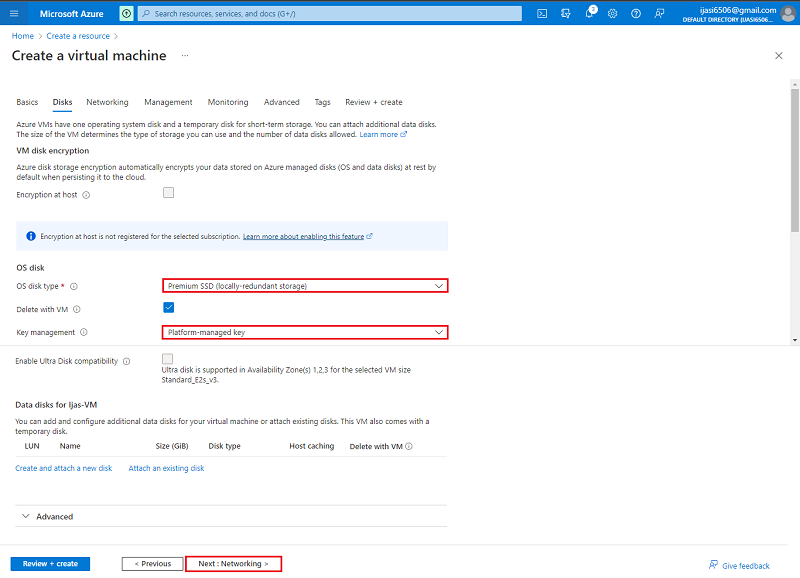In the image, we see the Microsoft Azure interface with the search field prominently displayed. The search field contains the placeholder text "Search resources, services, and docs." In the top right corner, the user's email, "ijaz6506@gmail.com," is visible alongside a "Default Directory" label. Several options are presented, including "Create a virtual machine," "Basics," "Disks," "Networking," "Management," "Monitoring," "Advanced," "Tags," and "Review + Create."

The caption also provides detailed information about Azure Virtual Machines (VMs). It mentions that VMs come with one operating system disk and a temporary disk for short-term storage. Additionally, users can attach more data disks as needed. It also highlights the security features of Azure's disk storage, noting that the virtual machine disk encryption and Azure disk storage encryption automatically encrypt the data stored on Azure managed disks. Both the operating system and data disks are encrypted at rest by default as they persist into the cloud.